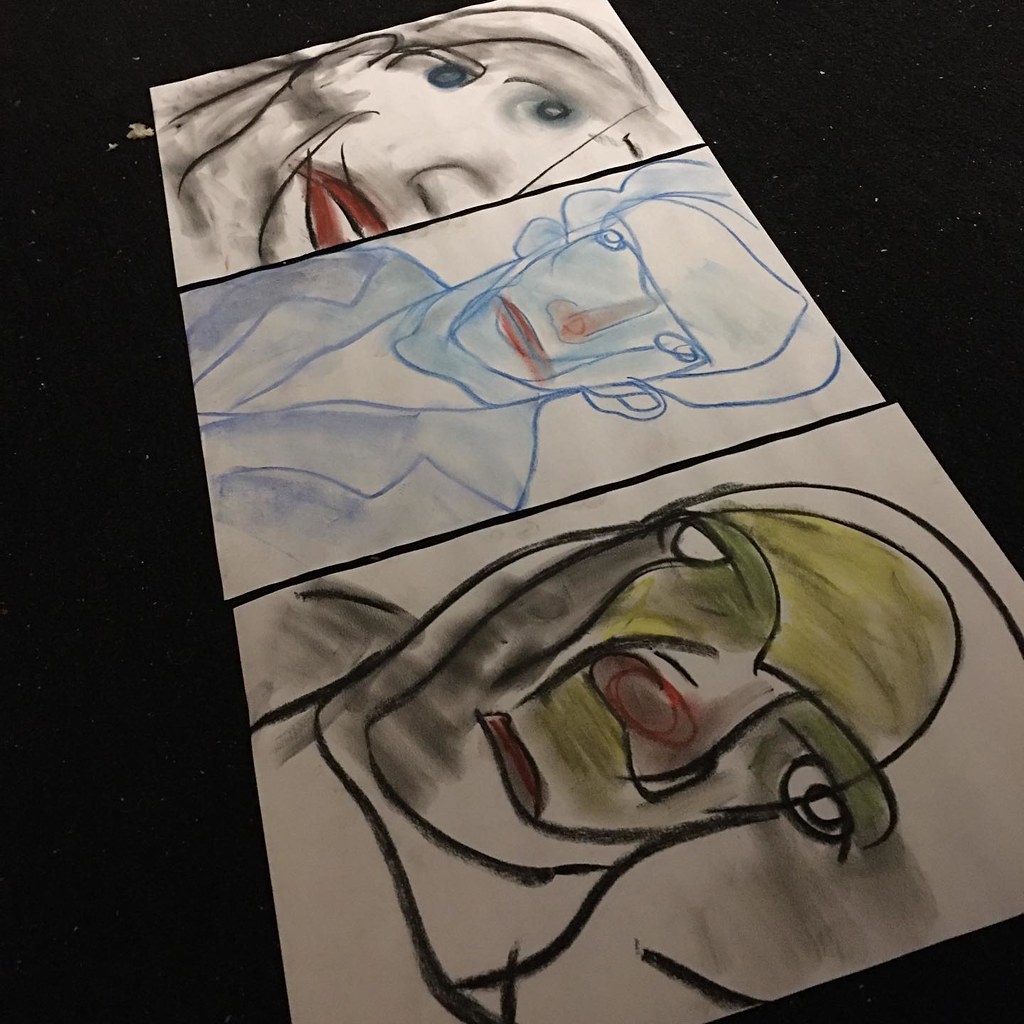This color photograph features a triptych of artwork arranged horizontally on a beige canvas, requiring the viewer to turn their head to the right for proper viewing. The three pieces are set against a black background with speckled details. 

The first piece depicts a minimalist line drawing of a person's profile, showcasing two bluish eyes and a prominent red mouth. The rest of the face is sketched lightly in pencil, with indications of longish hair framing the visage. 

The central artwork is a line drawing of a person's head and shoulders, predominantly outlined in blue. This figure has a red nose and mouth, and is clad in a blue jacket, minimally filled in with blue pencil, over a whitish top. 

The third piece steps into surrealism with a face drawn in black marker. The inner circle of the face is shaded light green, while the area between the eyebrows and the eyes is filled with a darker green. The nose edge and the thin mouth are accented in red, creating a striking contrast against the green and black elements.

This compilation of artistic expressions offers a unique juxtaposition of minimalism and surrealism, unified by their distinct use of color and line work.